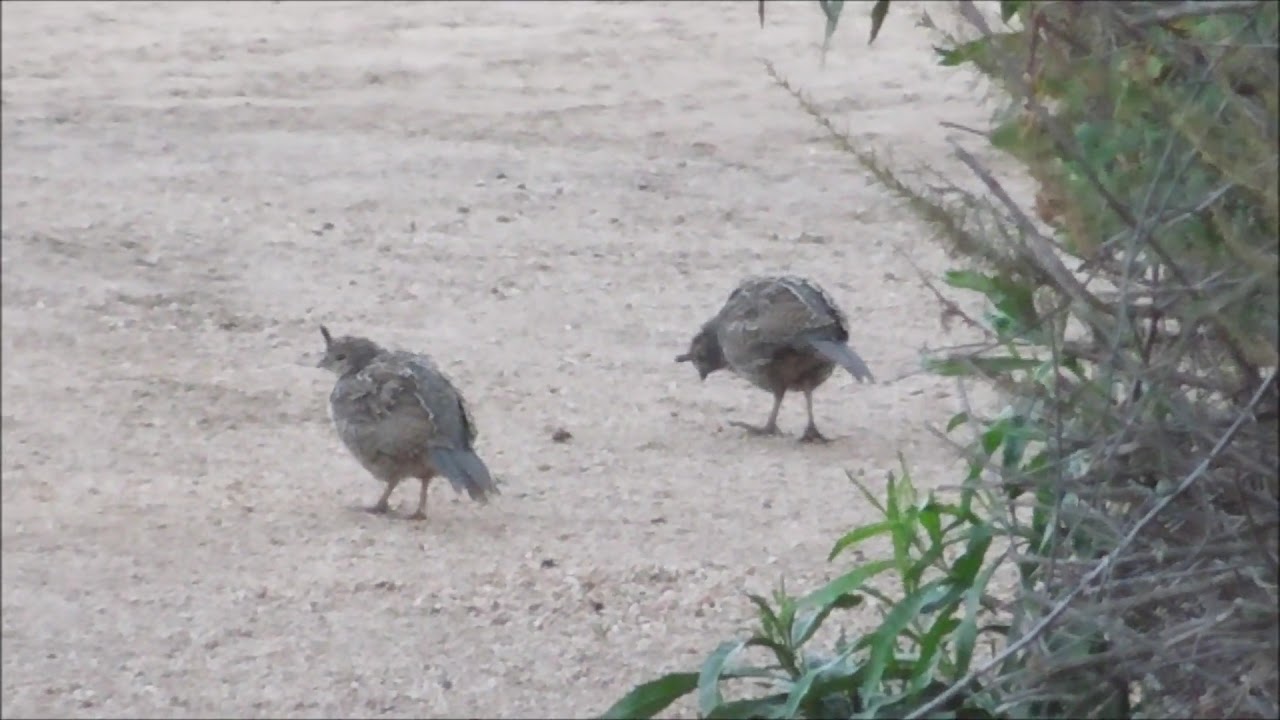This is an outdoor photo of two birds, likely quail, standing on a white surface that could be either concrete or sand, most probably concrete. The scene is set on an overcast day, evident from the dull background that lacks sunlight. The left side of the image is dominated by the birds, which are grayish with a hint of blue and brown legs. One bird is leaning over, pecking at the ground, while the other stands more upright, gazing towards the camera with an alert posture. On the right side of the photo, there is a mixture of vegetation: some brown, leafless branches and green, elongated bushes protruding from a border area. The surface beneath the birds is uneven, featuring various sized stones amidst the primarily brown color palette. Overall, the image captures a serene moment of these two birds exploring their environment for food.